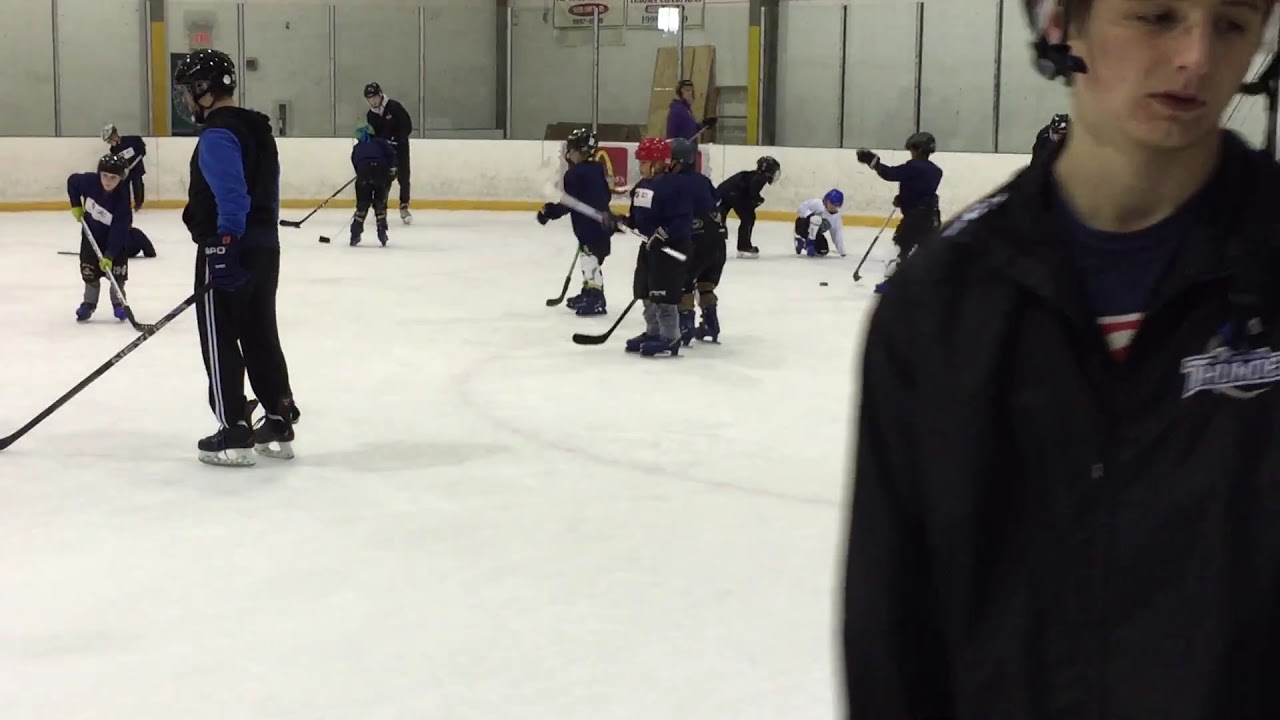The image captures a lively scene on an indoor ice rink, predominantly featuring children engaged in a game of hockey. Most of the children are outfitted in dark blue shirts, black shorts, and either blue or black skates, topped with black helmets. Notably, one child at the center stands out with a red helmet, while another child to the right, kneeling, sports a long-sleeve white shirt and a blue helmet. Amid the children, a few adults are present, including a man on the left dressed in a blue shirt with a black vest and black track pants with white stripes. The rink is pristine white with no visible markings, surrounded by a white wall with a yellow border at the base. To the far right, a person in a black shirt or jacket featuring a white logo that seems to spell "Thunder" is facing the camera, appearing somewhat somber with a headset on. Overall, the kids, centered on the ice, appear to be gearing up for practice, their movements and sticks suggesting the thrill of a hockey game in session. The setting exudes an indoor, mid-day ambiance, punctuated by the colors of their gear and the stark, clean environment of the rink.